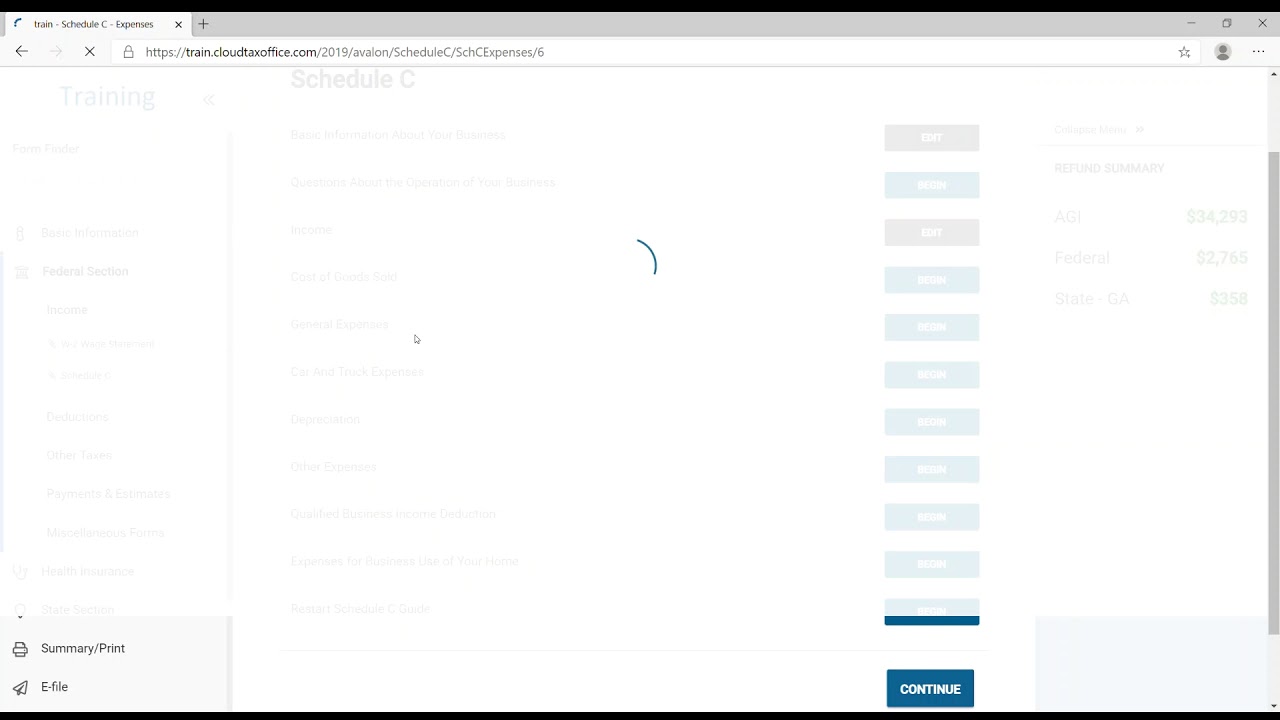This image captures a Google Chrome web browser with a gray theme, displaying a website used for text filing, specifically https://train.cloudtaxoffice.com. The main focus is on a semi-translucent overlay indicating content is loading, allowing visibility of the underlying page.

The visible elements indicate the user is in the midst of filing their taxes online. Prominently displayed is the refund summary, detailing an Adjusted Gross Income (AGI) of $34,293. The forecasted federal tax refund stands at $2,765, while the state refund for Georgia is noted as $358. Summing both, the approximate total refund amounts to around $3,123.

On the left side of the page, there is a navigation menu with sections for federal, income, summary, print, and e-file. The interface mentions "Schedule C," implying it’s for someone with business income. Each section contains editable subsections, with a visible “edit” button readily available. At the bottom of the page, a dark blue button labeled "Continue" in white text is present, guiding the user through the filing process.

This detailed depiction highlights the structured and user-friendly design of the text-filing software, ensuring ease of navigation and clarity in the online tax filing process.